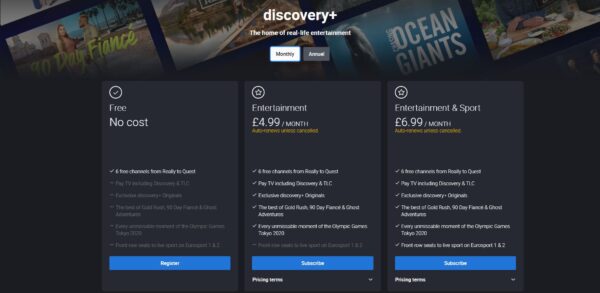The image is a screenshot from the Discovery+, a popular streaming service, as indicated by the Discovery+ logo prominently displayed at the top-center of the page. This specific screen appears to be the subscription selection page, offering users three distinct plans. 

On the left, the first option is the Free plan, which comes at no cost. The middle option, labeled as the "Entertainment" plan, is available for £4.99 per month. The third option on the right is the "Entertainment & Sport" plan, priced at £6.99 per month. 

Each plan includes brief descriptions of the content and features provided, positioned directly above their respective options. 

At the bottom of the page, beneath the subscription options, there is a prominent, elongated blue rectangle button for subscribing or registering for the service.

The background of the page is a sleek black, which enhances the visibility of the subscription details. 

At the top of the page, serving as a header, are thumbnail images of featured content available on Discovery+, including titles like "Ocean Giants" and "30 Day Fiance."